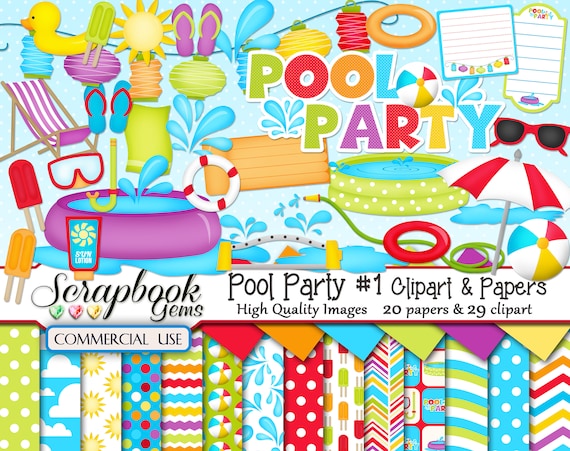The image is a highly detailed, vibrant cover for a scrapbooking book titled "Scrapbook Gems: Pool Party". The cover is a medley of colorful graphics and text, predominantly featuring a blue background with white polka dots. At the top, in playful, colorful text, it reads "Pool Party" with splashes of blue water symbols surrounding it. Below, written in black cursive, "Scrapbook Gems" introduces the book's theme, followed by a blue rectangle containing the text "Commercial Use". 

The middle section of the cover elaborates on the book’s content: "Pool Party, Number One Clip Art and Papers, High Quality Images, 20 Papers, and 29 Clip Art". Surrounding this text are various pool-themed clip art illustrations such as sunglasses, a beach umbrella, flip-flops, a beach ball, sunscreen lotion, inner tubes, and a rubber ducky. Brightly colored hearts shaped like gems (green, pink, and yellow) also add to the playful vibe.

The lower half showcases an array of patterned scrapbook papers presented in small strips. These include designs like green with white polka dots, blue with clouds, white with sunshines, blue with multicolored polka dots, white with wavy colored lines, white with blue splash watermarks, red with white polka dots, and several others with various playful patterns, such as beach balls, popsicles, and more "Pool Party" themed designs.

In the center left side, additional colorful illustrations further emphasize the pool party theme, including a beach chair, a purple swimming pool, suntan lotion, and water splashes, while on the far right side, "Pool Party" with lines to write words appears, highlighting the book's usability for personalized scrapbooking projects. The overall presentation is lively, engaging, and evokes summer fun, making it an attractive resource for scrapbooking enthusiasts.